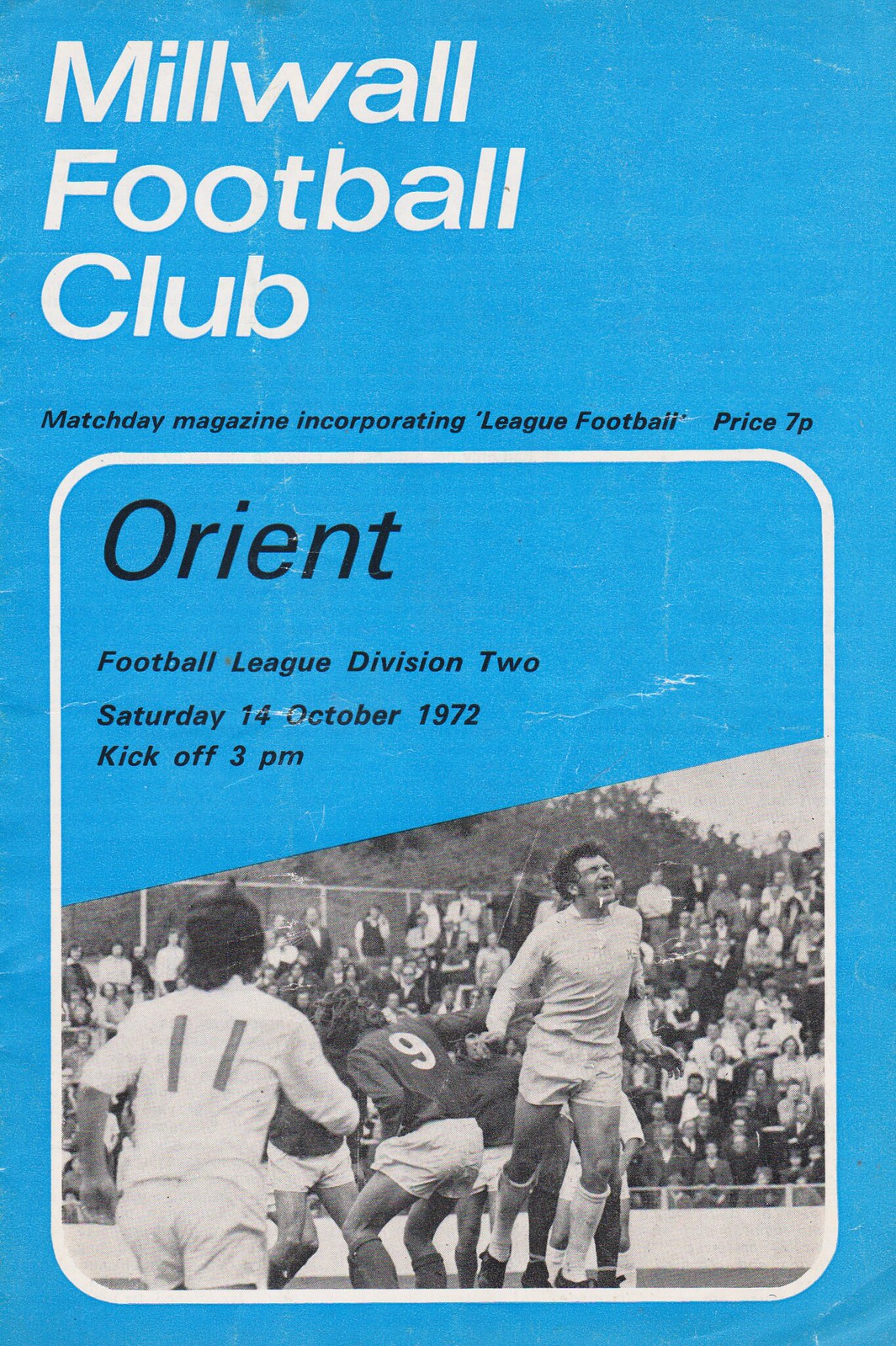This image features a vintage cover of the Millwall Football Club Match Day Magazine, dated Saturday, 14th October 1972, for a Football League Division Two match. The cover is set against a sky blue background and is arranged in a portrait orientation, making it taller than it is wide. At the top, bold white text proclaims "Millwall Football Club," with smaller black text below it stating "Match Day Magazine Incorporating League Football" and listing the price as 7p, presumably pence, a UK currency. Beneath this, a white-bordered rectangular box contains additional details about the match: "Orient Football League Division Two, Saturday, 14th October 1972, kickoff at 3pm."

Inside this white-bordered box, the bottom half includes a black-and-white photograph capturing a moment from a soccer game. The players are intensely focused on the game, while a sizeable crowd of spectators fills the stadium seats in the background. One player's face is distinctly visible as he turns towards the camera, adding a touch of human interest to the historic scene. This blend of textual and visual elements creates a nostalgic snapshot of a football match from the early '70s.